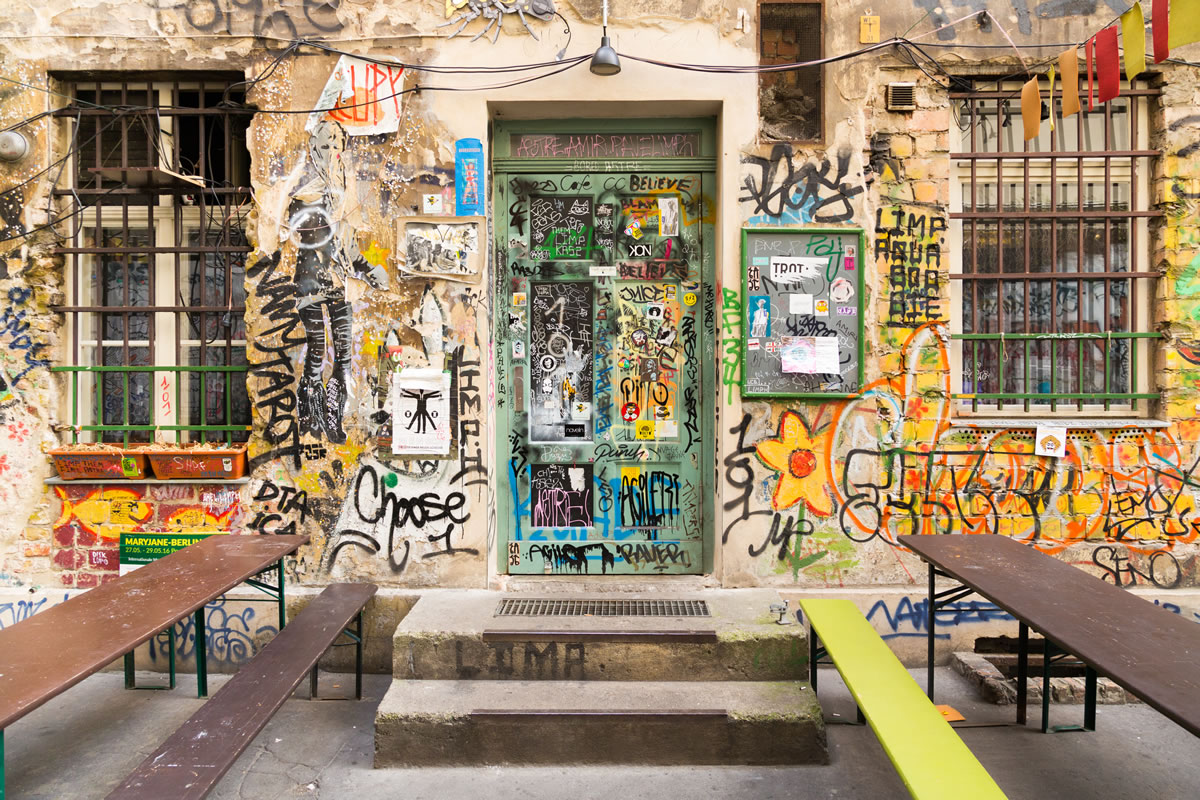The image depicts the front of an old, possibly abandoned building, heavily adorned with graffiti in a myriad of colors including black, blue, white, green, pink, and orange. The building, constructed of bricks and cement, features a light orange or beige stucco façade that is extensively vandalized. Dominating the center is a greenish door, almost entirely obscured by graffiti, intricate writings, and drawings. Notable tags include "Chase," "Limp," "Barbie," "Madjarst," and "D.T.A." Above the door, exposed wiring and a hanging lamp can be seen. The entrance is flanked by two multi-pane windows, secured with bars that are green at the bottom and brown at the top.

At the base of the building, two concrete steps, marked with black graffiti including the word "Lima," lead up to the door. There's also a brown metal grate at the top of the steps. On either side of the entrance, there are picnic-style benches—on the left, a light brown wooden bench supported by green steel beams, and on the right, a table with a gray top and a greenish-yellow seating area.

The scene is set in bright daylight, and multiple layers of graffiti across the walls and door suggest that the building is not in regular use. Additionally, a line of colorful flags, starting with yellow and red and spanning multiple colors, adds to the visual chaos. The setting and the extensive graffiti give the impression of an old, possibly neglected storefront that has become a canvas for street artists.